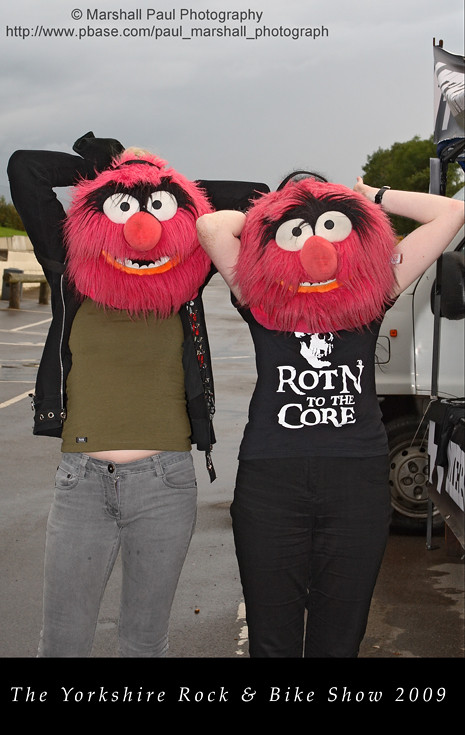The image captures a gray, overcast day with a wet sidewalk, possibly after a recent rain. It features two women standing with their arms raised and bent behind their heads, each wearing a red furry Muppet-like mask. The masks have toothy grins, bushy black eyebrows, googly white eyes, and big, orangey-red noses. The woman on the right is dressed in black jeans and a black T-shirt that says "Rotten to the Core" with a skull design, while the woman on the left wears dark, faded jeans, an olive-green T-shirt revealing some midriff, and a black jacket with silver detailing. Behind them, a white truck is partially visible to the right, and another truck can be seen further down the road to the left. The top of the image is branded with "Marshall Paul Photography" and a website link, while the bottom features a black banner stating "The Yorkshire Rock and Bike Show 2009."